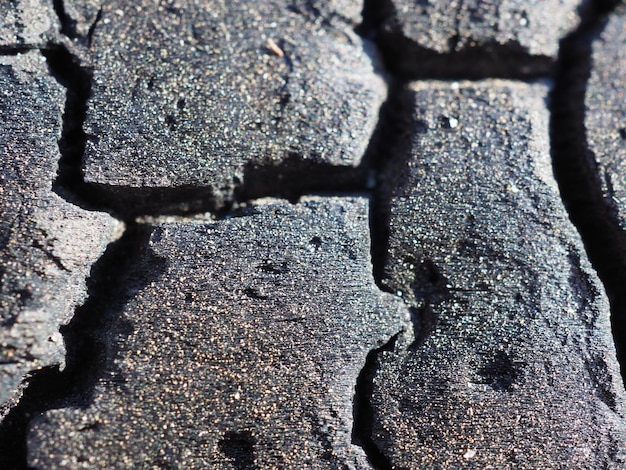A square, close-up, full-color photograph depicts a section of an outdoor stone walkway or wall on a sunny day. The dark gray stones, varying in size and shape, are interconnected but appear fragmented by deep, dark black channels that signify cracks or separations. The stones exhibit a rich texture, featuring concavities, fine horizontal lines, and occasional divots. The surfaces of the rocks are speckled with light gray, brown, yellow, and very light sage green flecks. The arrangement of the stones is irregular and jagged, highlighting a natural or handcrafted pattern that creates a mosaic-like effect. Shadowing enhances the monochromatic theme of the detailed, textured scene.